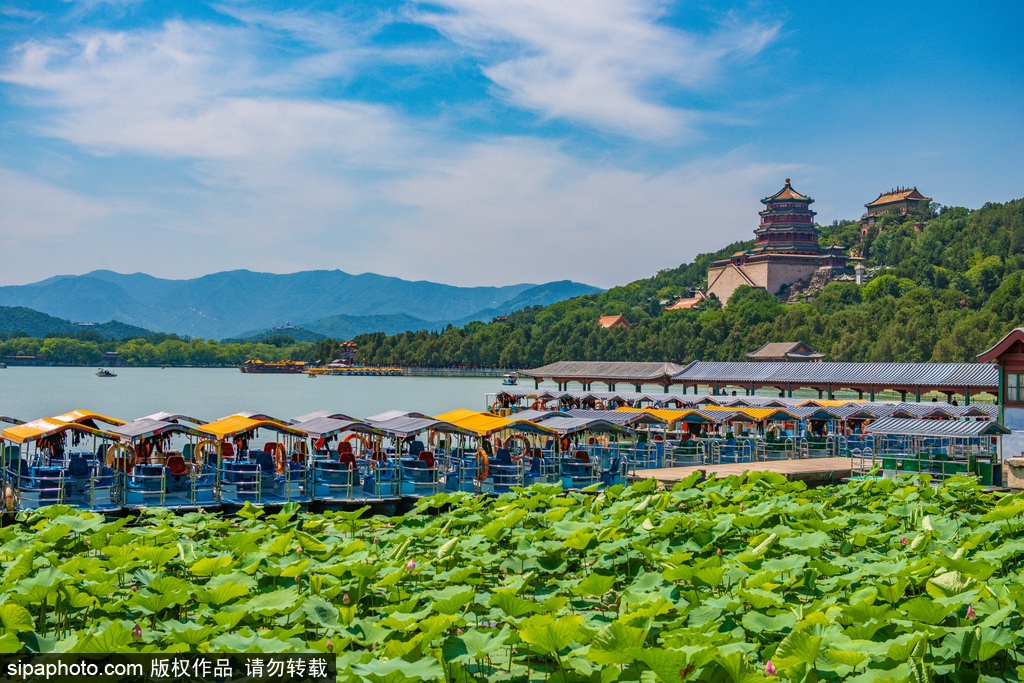This image captures a serene lakeside scene, likely from an Asian tourist location, bathed in sunlight under a clear blue sky with wispy white clouds. Dominating the background are dark gray hills, while dense green trees carpet the slopes closer to the lake, which occupies the foreground. On the right, the hills ascend, revealing a distinctive light brown structure that resembles a monastery with a square base and a central cylindrical portion topped by a triangular roof. Directly in front, vibrant green shrubbery frames the scene, adding a lush contrast to the blue water.

The lake is dotted with long, flat-roofed boats featuring blue seats, likely catering to tourists. More colorful boats, both large and small, float on the water, suggesting a mix of traditional and modern designs, possibly including mechanical skimmers. To the bottom left of the lake, large lotus-like plants and flowers spread across the water surface. At the bottom left of the image, a red box contains the text "seepaphoto.com" in both English and Chinese characters, solidifying the photograph's likely Asian heritage.